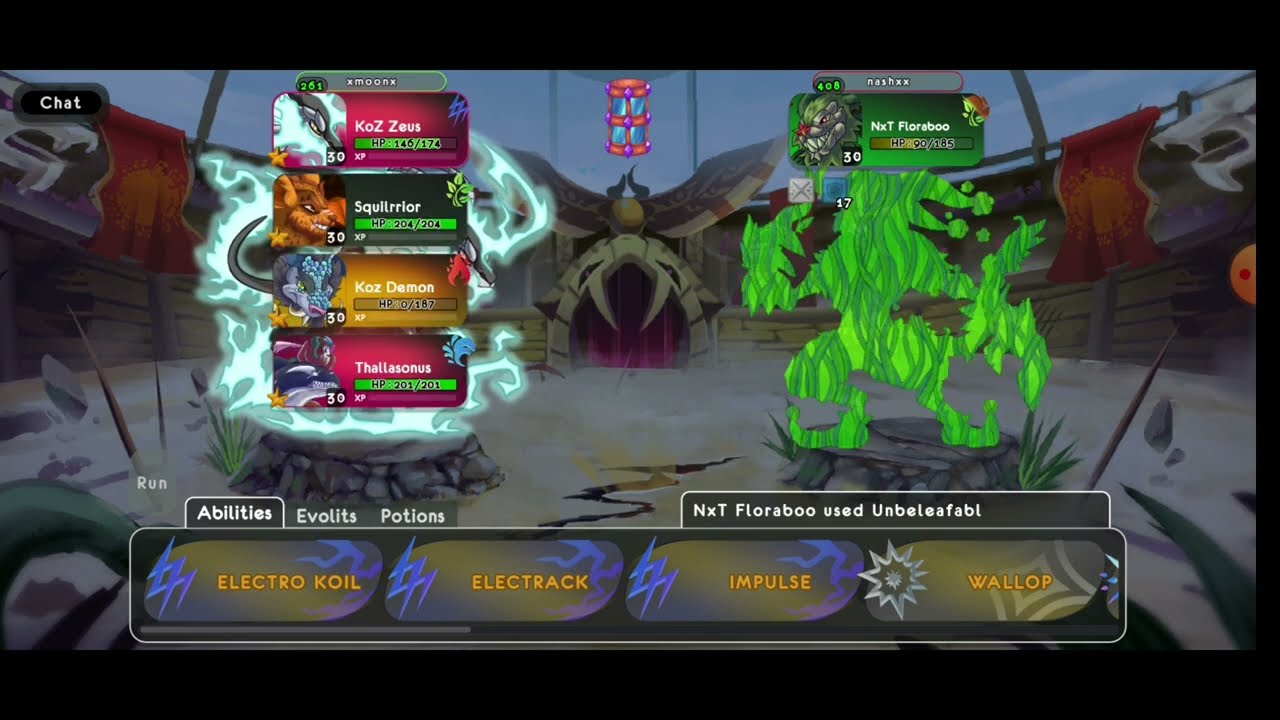This is a detailed screenshot of a video game featuring a fantasy battle scene involving dragons. The image has a thick black border at the top and bottom, and a thinner black border on the right side. The background depicts a dome-like structure with a gold archway and a red door in the middle, flanked by two fangs. The top portion of the dome is glass. In the top left corner, there is a black bubble displaying a chat section. The right side of the image shows a green dragon character from player Nash_xx, who is winning with a score of 408. The left side features a bluish-black dragon character from player Xmoon_x, who has a score of 261. Both dragons appear to be standing on rocks in a body of water, and the scene is set in a rounded stadium or enclosure. Four different colored icons with animal or character images are positioned above the dragon on the left. At the bottom of the screenshot, there are four squares within a long rectangle, labeled with different abilities: Electrocoil, Electrac, Impulse, and Wallop. Another tab reads "NXT Floral Boo used Unbelievable," and further text displays "evil it's" and "potions."